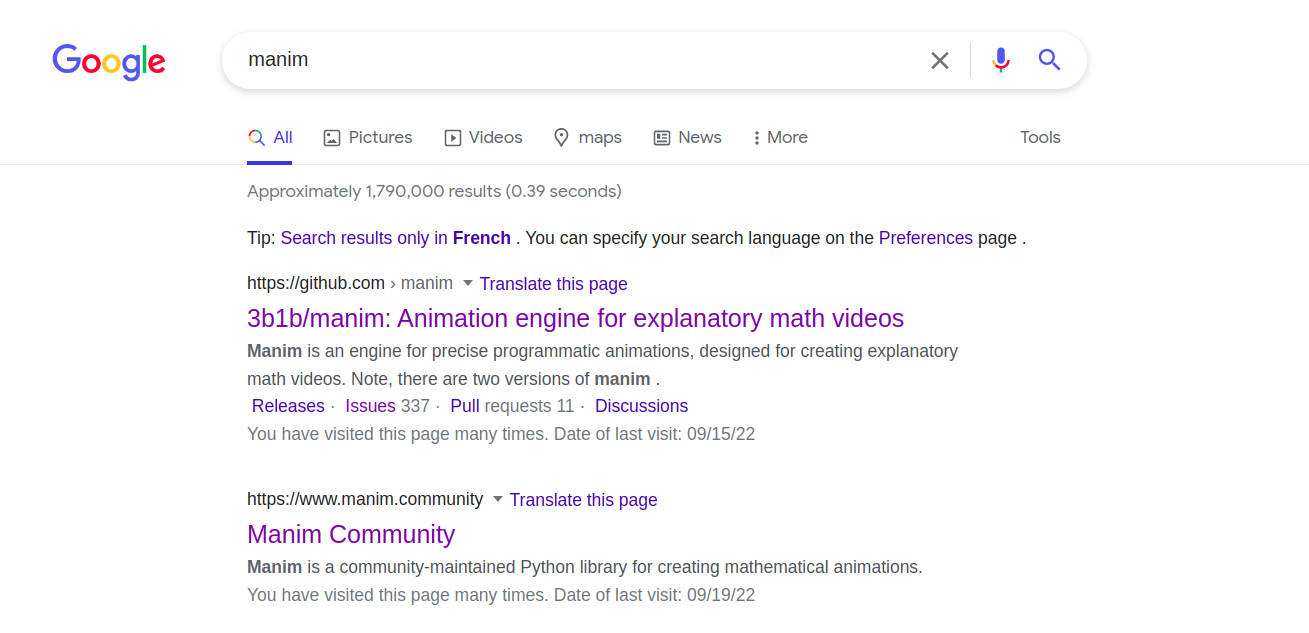A voice search for "Manim" yields approximately 1.79 million results. Users are advised that they can specify their search language on the preferences page, with a tip suggesting they can narrow down to results in French. The first result, hosted on GitHub under the repository named "3b1b/Manim," describes Manim as an animation engine for creating explanatory math videos. The second result leads to "Manim.community," identifying Manim as a community-maintained Python library for generating mathematical animations. Both listings likely refer to the same software tool, used by the popular YouTube channel "3Blue1Brown," renowned for its clear explanations of complex math and science topics. For context, this screenshot has a white background.